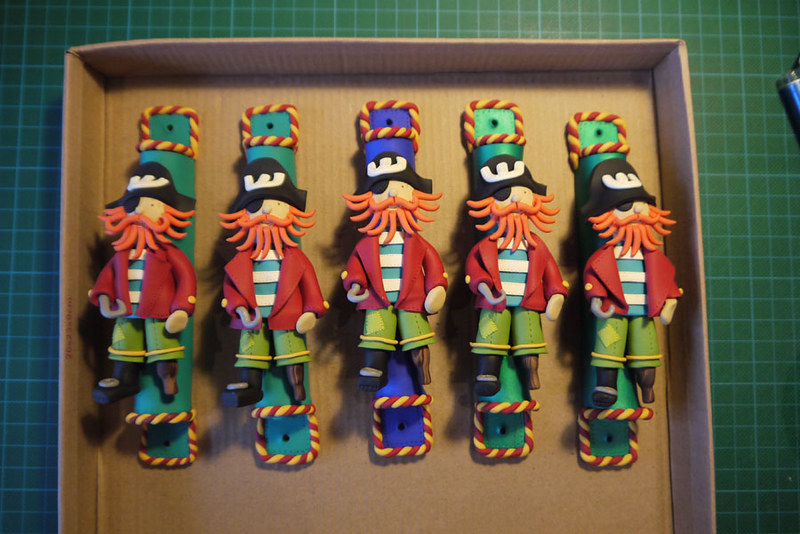The photograph captures five colorful pirate figurines, intricately crafted and housed in a brown cardboard box. The background resembles a thick green rubber cutting mat, patterned with white grid lines akin to graph paper. Each pirate figurine has notable, uniform features: dressed in blue and white striped shirts beneath red jackets adorned with yellow buttons, light green pants with yellow trim, a black eyepatch covering the right eye, and a distinctive black pirate hat marked with a white 'W.' They sport red beards and mustaches, each bearing a silver hook on their right arm and a wooden peg for the left leg, complemented by a black boot on the other leg. Mounted on multicolored holders—ranging from light green to blue—they appear ready for display, possibly as handmade toys or wall hangings. The craftsmanship suggests a meticulous and detailed art project, perhaps fashioned from clay, highlighting the whimsical and consistent design of each pirate figure.